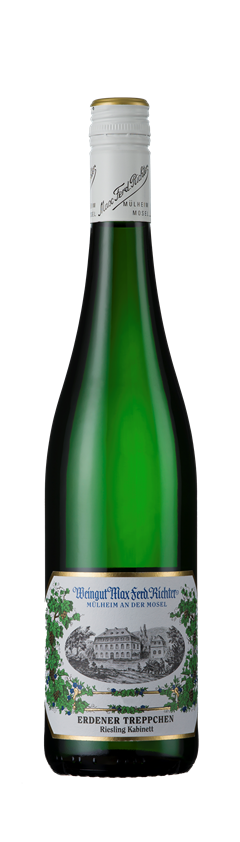This image features a green glass bottle, likely containing some type of alcoholic beverage, floating against a plain white background. The bottle is cylindrical with a long, narrow neck that is closed with a gold and white cap. Around the neck, there is a white label featuring black cursive text, though the lettering is not entirely legible. The bottle's main label, positioned near the base, has a striking gold border and a white background.

Centrally placed on the label is a detailed black-and-white illustration of a large mansion, surrounded by vegetation. Flanking this illustration, on both the left and right sides, are decorative green leaves and vines. Above the image, in blue text, the title includes the word "Weingut," likely part of the name "Weingut Max Ferd. Richter." This text is followed by the locations "Molheim" and "Mosel," indicating the geographic origin of the beverage. Below the central illustration are two lines of black text, providing additional descriptions, one of which notes "Erdener Treptchen, Riesling Kabinett," with "Kabinett" distinctly spelled.

Overall, the bottle's design and labels suggest a sophisticated product, with meticulous attention to aesthetics and detail, reflective of its presumably high-quality contents.